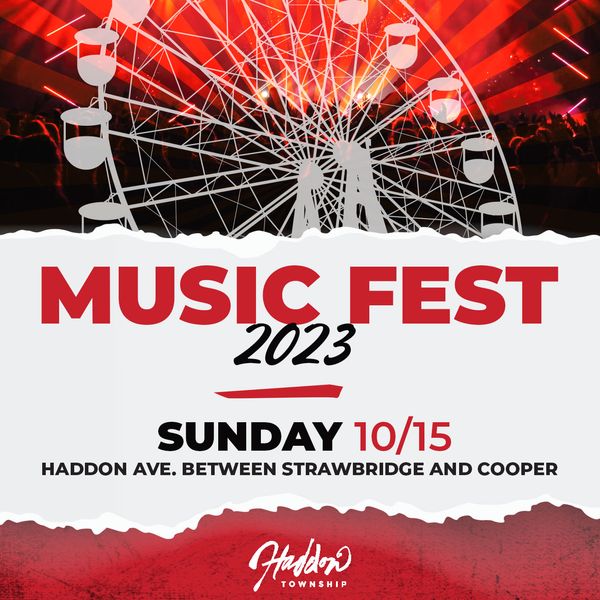The poster features a vibrant and striking design in red, white, and black. At the center, amidst a white background with jagged, curvy edges, large red capital letters announce "MUSIC FEST." Directly beneath, the text "2023" is written in black italics, underscored by a bold red line. Below this, the word "SUNDAY" appears in black capital letters, followed by "10/15" in red, denoting the date of the event in a slightly smaller font.

Further down, detailed logistical information is provided in black capital letters: "HADDON AVE. BETWEEN STRAWBRIDGE & COOPER." The bottom of the poster is framed with a jagged red border, and the text "HADDON TOWNSHIP" is prominently displayed in white at the footer.

The upper third of the poster features a stylized depiction of a Ferris wheel in white, set against a dynamic backdrop of black and red streaks creating a sunburst effect. The entire design is bold, energetic, and clearly communicates the essential details and excitement surrounding the Music Fest event.